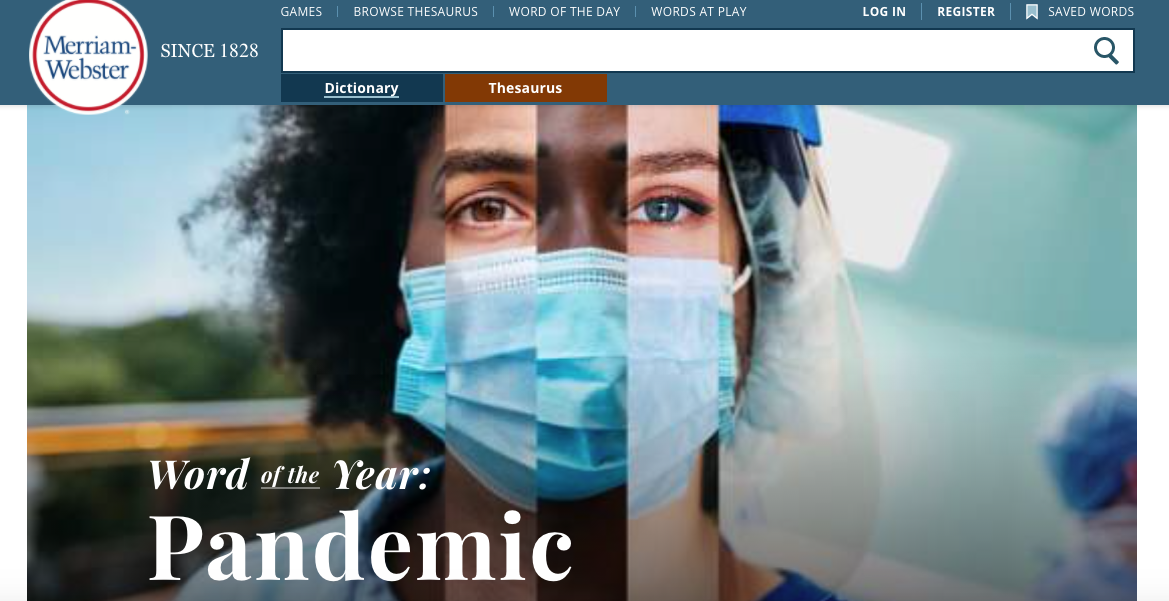The image is a screenshot of the homepage of the Merriam-Webster website. At the top-left corner, there is a prominent white circle containing the text "Merriam-Webster." To its right, the phrase "Since 1828" is displayed. Across the width of the page, spanning from the left to the right side, is a large search bar. Directly below the search bar are two navigation categories labeled "Dictionary" and "Thesaurus."

The central portion of the homepage is dominated by a collage featuring five individuals, each wearing a protective blue face mask. This visual element emphasizes the widespread impact of health precautions in recent times.

Toward the bottom left side of the page, there is text that reads "Word of the Year." Beneath this, prominently displayed in larger white letters, is the word "Pandemic." This stark, bold font underscores the significant influence the term has had over the past year.